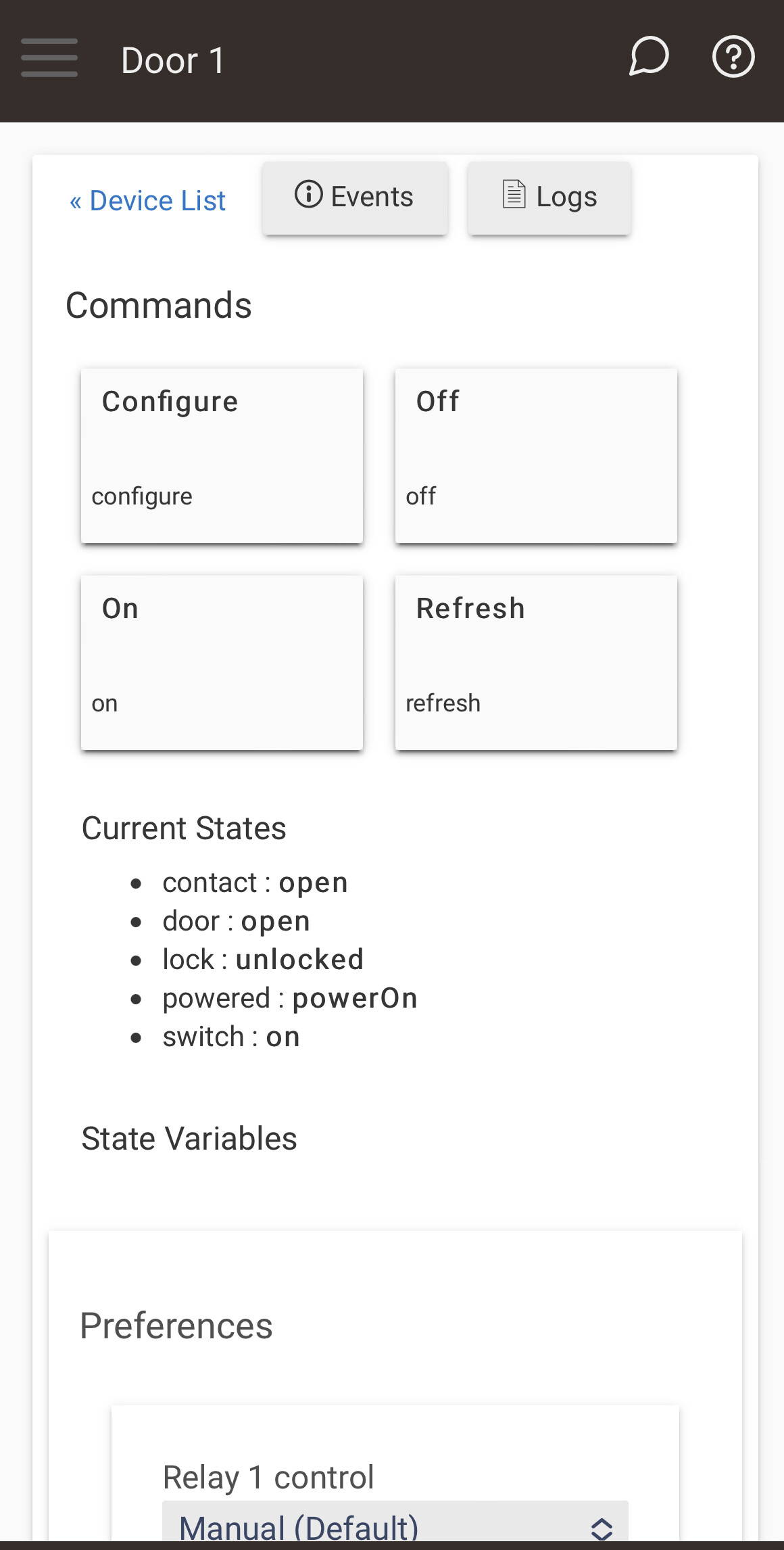This detailed screenshot showcases a user interface with a clean and organized layout:

At the top of the interface, there are three light brown horizontal lines serving as a header. Written in white text over a brown background within this header is "Door 1". Below this header, there is a message bar accompanied by a circle icon with a question mark inside it, likely for help or additional information.

The main section of the interface is divided into several distinct areas. First, there are two white-background boxes with slightly off-white backgrounds inside, labeled "Event Logs" in brown text and "Device List" in blue text. 

Further down, there are four shadowed boxes giving the illusion of depth. These boxes are prominently labeled "Commands" and include options for "Configure", "On", "Off", and "Refresh". Additionally, the status of various components is displayed, such as "Current Status", "Contact Open", "Door Open", "Lock", "Unlock", "Power", and "Power On".

Moreover, there are interactive elements for controlling devices with statuses like "Switch On". Towards the bottom, there's a section labeled "State Variables" followed by a box named "Preferences" showing a version number "Relay 1.12". Lastly, an option for "Manual Default" is provided, ensuring comprehensive control over the system's settings.

This detailed and systematic layout facilitates efficient user interaction and real-time monitoring of the system's status.